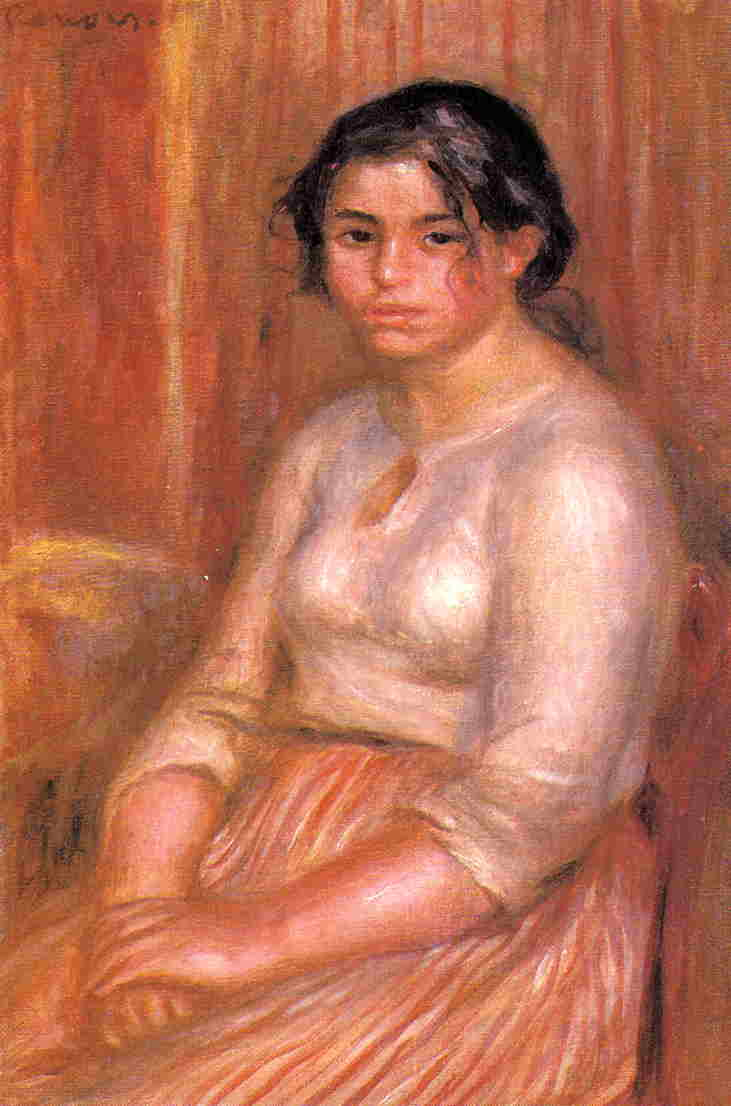This is a detailed painted portrait of a young woman with dark, tied-back hair that’s slightly frayed in the front. She has a thin face, a thin nose, and is noted to have a thick neck and broad shoulders for a female; she appears somewhat chubby. The woman is wearing a white, flowy top paired with a silky, pleated skirt that appears to be red or pinkish-peach. Her posture is relaxed as she sits slouched slightly forward in a chair, her right hand resting on her lap with her left hand gently placed over it. She gazes directly at the viewer, exuding a sense of calm. The background is a blend of monochromatic hues—red, orange, peach, with a touch of yellow—rendered in a painterly style with visible lines on the walls. The somewhat blurred background contrasts with the detailed depiction of the woman, enhancing her prominence in the composition. There is a signature in the top left corner, emphasizing the artistic nature of the portrait.